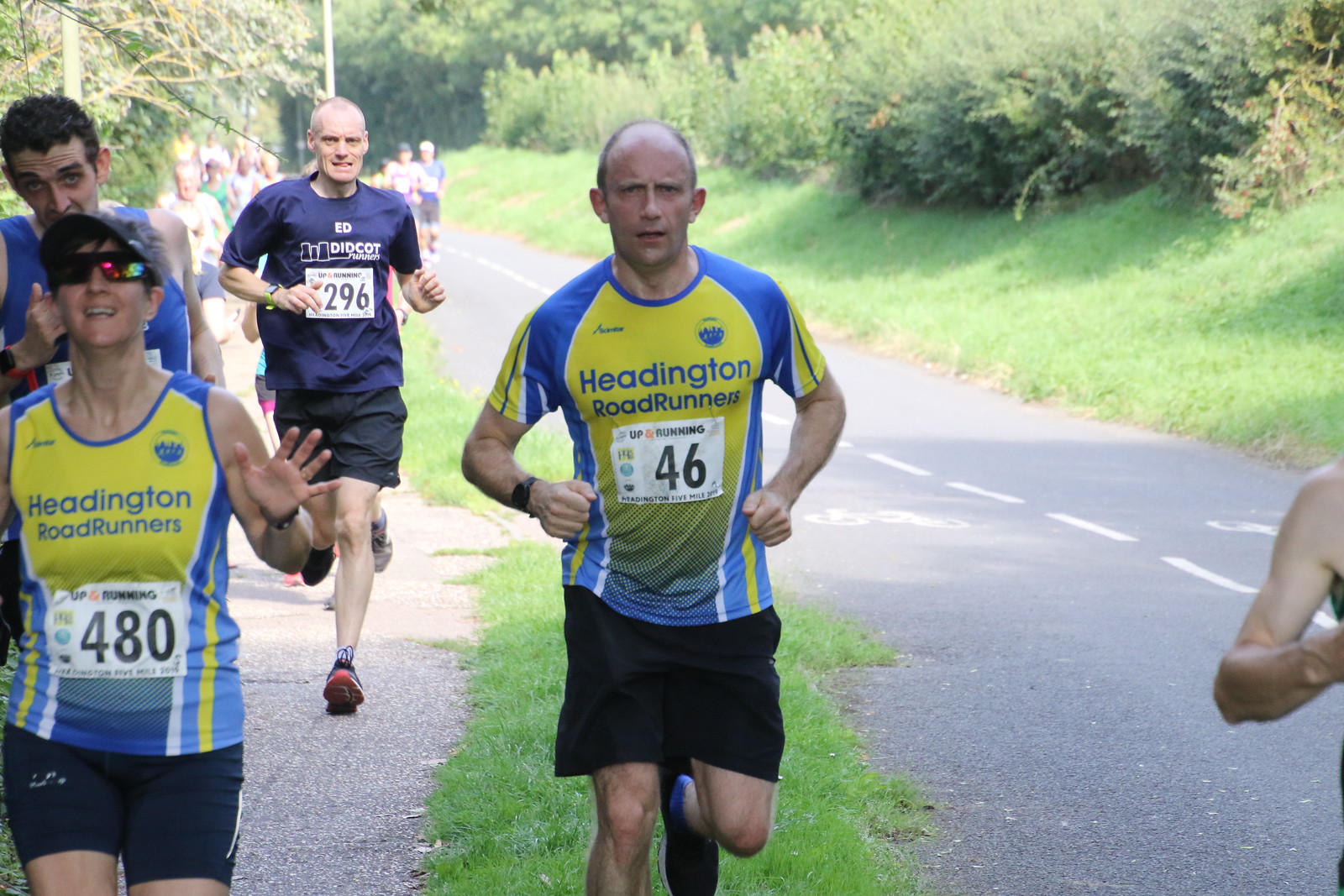The image captures a vibrant marathon taking place on a narrow bike path that resembles a small country road winding through a lush, forested area, possibly a national park. The setting is sunny and the path is bordered by green grass and trees. Central to the scene are the two lead runners: a balding man in his 40s and a woman next to him, both sporting yellow and blue jerseys with blue stripes and checkered marks that read "Heddington Road Runners." The man wears the number 46, while the woman, who is smiling at the camera in sunglasses and a blue hat, wears the number 480. Just behind them, a serious-faced older man dons a blue t-shirt with "Ed Didcot" and the number 296, paired with black shorts. More runners can be seen in the background, adding to the lively atmosphere of the race.